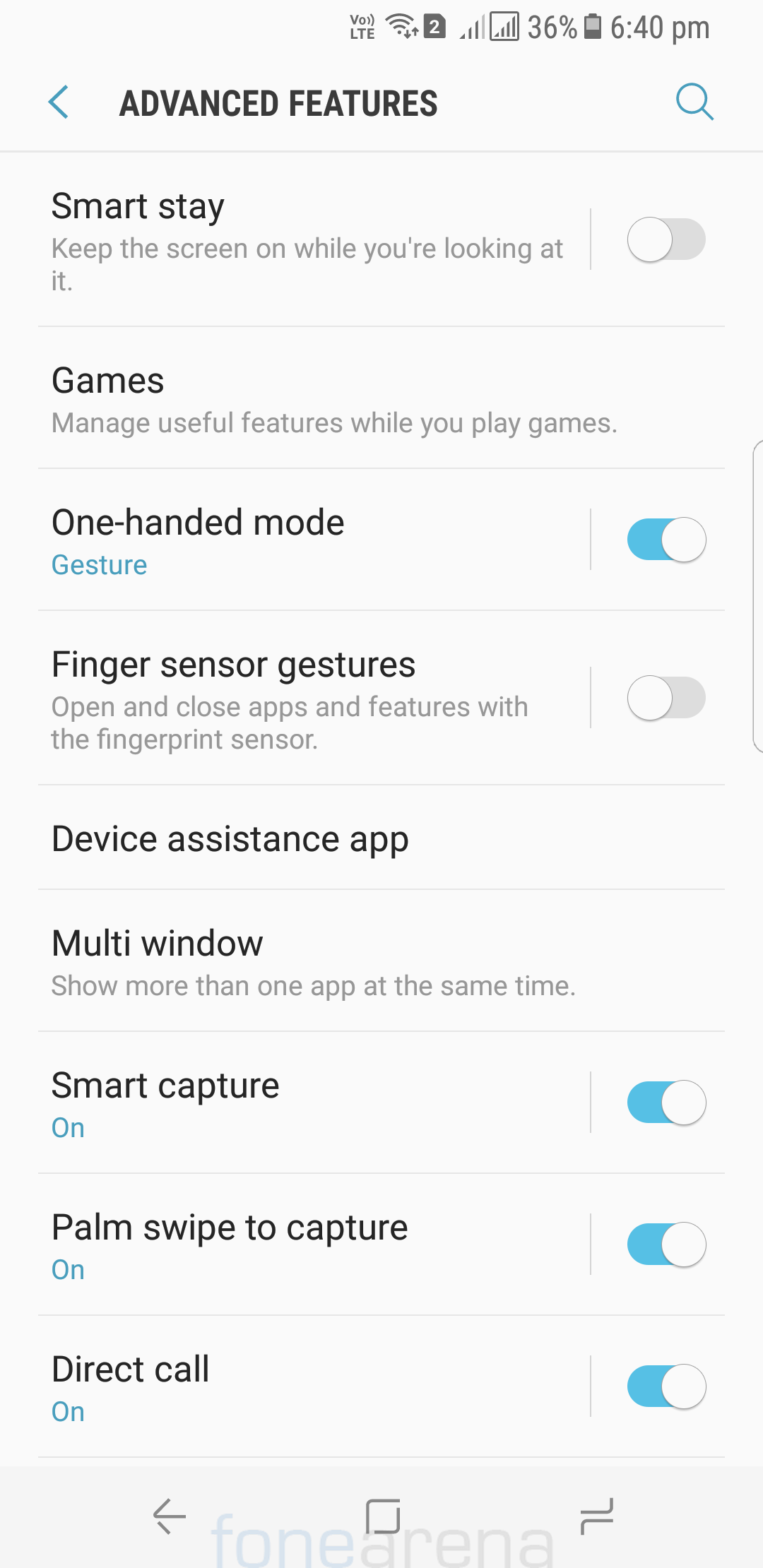The image showcases the Advanced Features panel on a smartphone. It’s currently 6:40 p.m., with the battery level at 36%, and the device connected to Wi-Fi. At the top of the display, the heading "Advanced Features" is prominent. The panel lists various settings as follows:

1. **Smart Stay**: Keeps the screen on while you are looking at it; this feature is toggled off.
2. **Games**: Manages useful features during gameplay.
3. **One-Handed Mode**: Enables gesture controls for one-handed use; this feature is toggled on, indicated by a blue-colored switch.
4. **Finger Sensor Gestures**: Allows the use of the fingerprint sensor to open and close apps and features; currently toggled off.
5. **Device Assistance App**: Settings related to device assistance apps.
6. **Multi-Window**: Allows viewing more than one app simultaneously.
7. **Smart Capture**: Enabled, facilitating advanced screen capture features.
8. **Palm Swipe to Capture**: Also on, allowing screen capture via a palm swipe gesture.
9. **Direct Call**: This feature is active, enabling the phone to call a contact when you bring it close to your ear.

Each feature is distinctly listed along with its current status, providing an insightful overview of the device’s advanced functionalities.